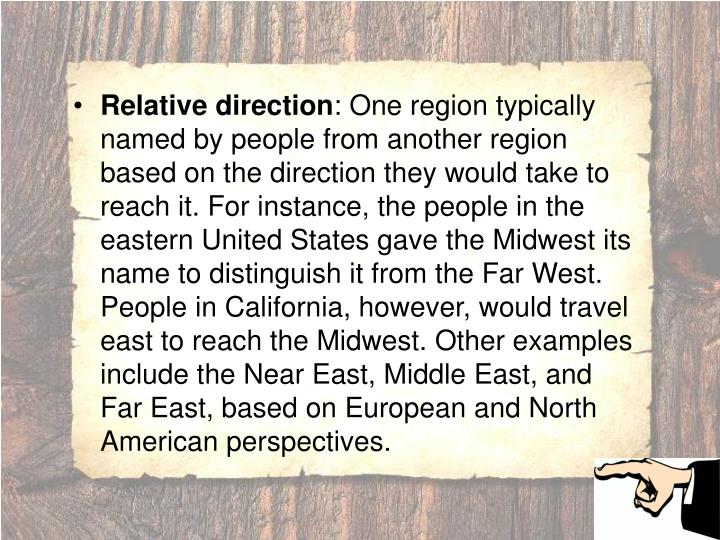The image depicts an educational presentation slide featuring detailed text against a background that resembles the grain of a wooden surface with gray and light brown vertical stripes. Centered on this background is a white sheet of paper with distressed, torn edges and a single black bullet point in the upper left corner. The text is left-aligned and describes the concept of "relative direction," explaining how regions are named based on directional perspectives. For instance, the Midwest was named by people in the eastern United States to distinguish it from the Far West, whereas Californians would travel east to reach the Midwest. Additional examples such as the Near East, Middle East, and Far East are also mentioned. The text spans 11 lines and is written in bold. In the bottom right corner of the image, a finger wearing a black sleeve points towards the text, reinforcing the educational and possibly slide-based nature of the presentation. The overall palette includes shades of brown, yellow, black, white, and light peach.